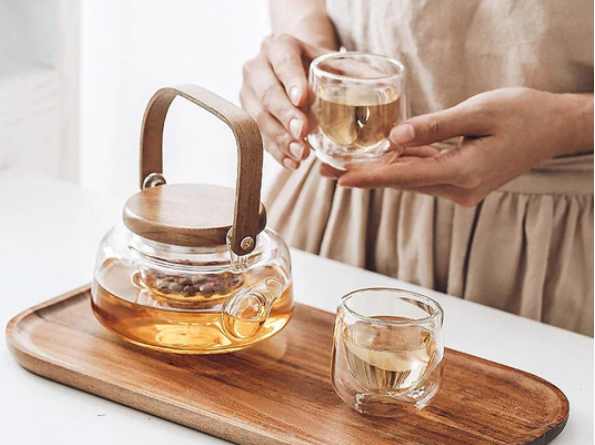A woman, possibly of Indian descent, with an olive complexion, is standing in a brightly lit kitchen. She is wearing a beige dress or apron and holding a clear glass filled with golden jasmine tea. In front of her, on a pristine white countertop, there is an elongated rectangular wooden tray. This tray holds a clear glass teapot with a wooden handle and lid, containing jasmine tea. Beside the teapot, there is another clear glass filled with the same golden liquid. The soft light flooding the background adds a serene and inviting ambiance to the scene.